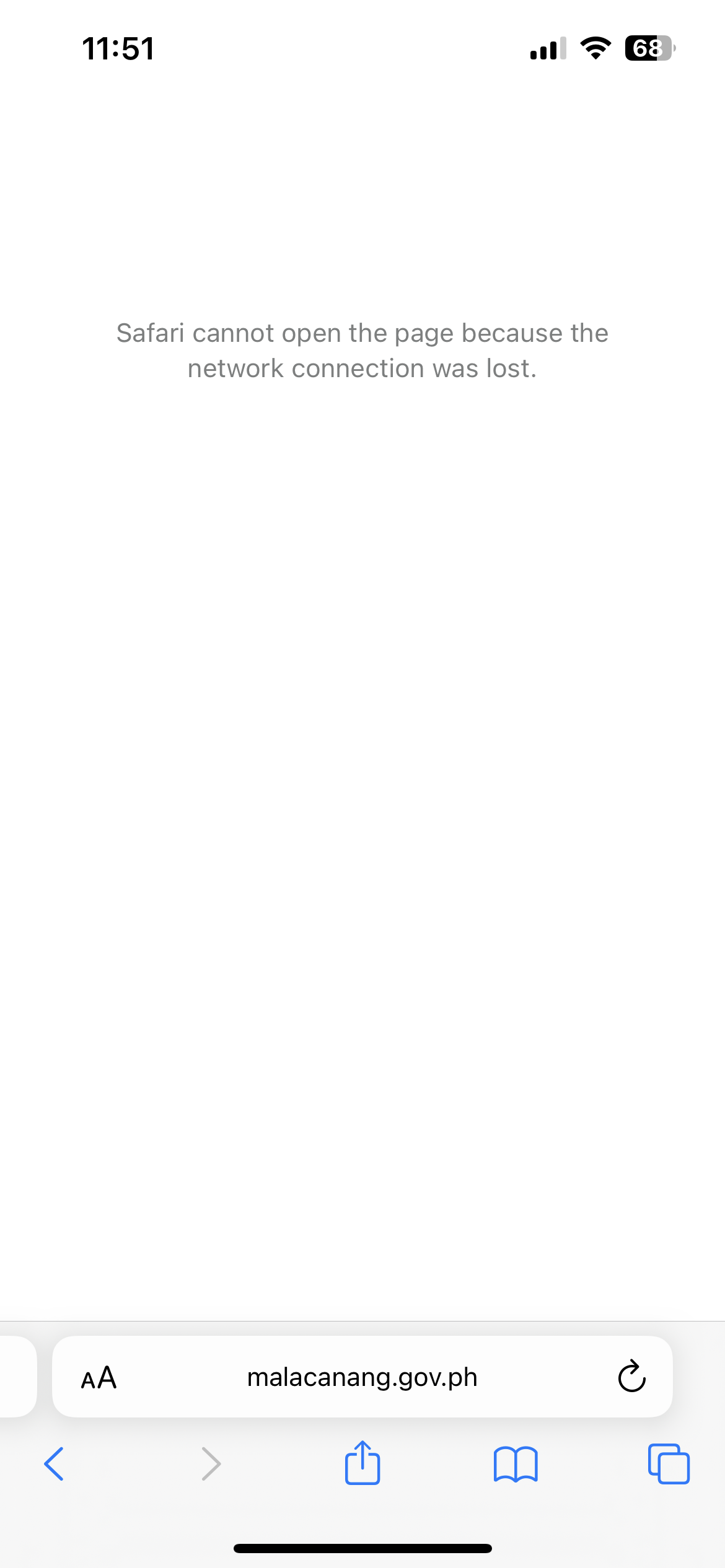A screenshot captured from a mobile phone at 11:51 AM displays the current status of the device. The signal strength is robust, and the battery stands at 68%. The background of the screen is predominantly white, accented by light gray text. The message, rendered in gray lettering, reads: "Cannot open the page because the network connection was lost." 

At the bottom of the screen, user interface elements include a small capital 'A' and a larger capital 'A' positioned in a white box against a gray background, indicating adjustable text sizes. Adjacent to this box is the text "malakeninga.gov.ph," alongside a refresh icon.

Below these elements are several navigation icons: a blue left-arrow for backward navigation, a gray right-arrow for forward navigation, and a series of blue icons representing different functions. These include an upward-facing arrow within a page icon, a split-page icon, and an overlapping two-page icon. These elements indicate various in-app actions possibly related to navigation, sharing, or viewing options. The overall interface suggests the user was trying to access a webpage but was hindered due to a lost network connection.